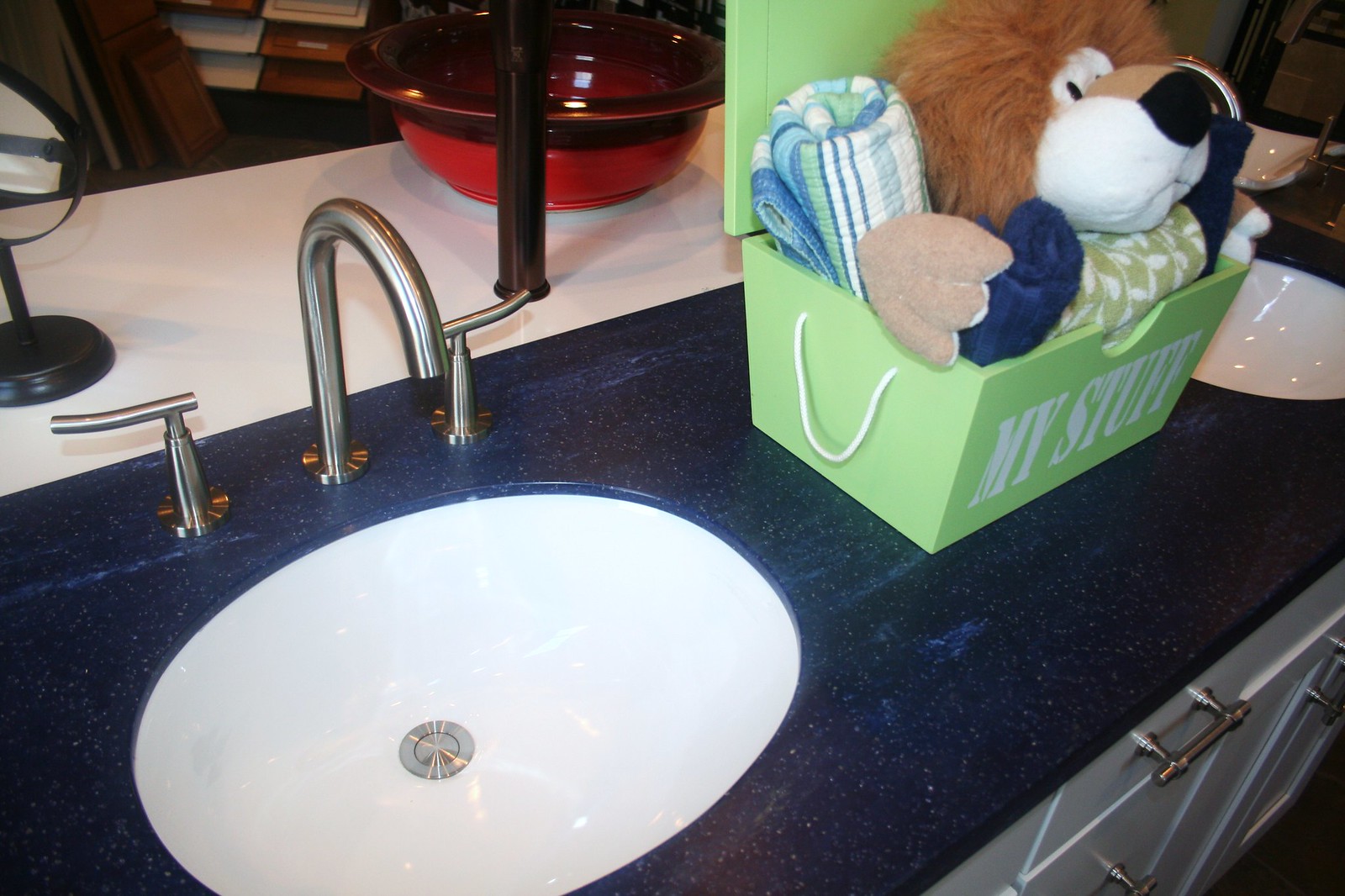The image showcases a bathroom scene featuring a double sink setup. The countertops have a bluish hue with flecks of white. In between the two sinks, there's a green box labeled "My Stuff" containing various items. Among these are a rolled-up green towel, a blue towel, and a multi-colored towel in shades of white, blue, and green. Also in the box is a stuffed animal resembling a lion. 

The right-side sink is white with a center section that prevents water from draining. It is equipped with a modern silver faucet and separate hot and cold handles. Beneath the sink are white cabinets fitted with steel handles. The floor, although slightly out of focus, appears to be brown.

In the background, there's a red bowl and a mirror with a black frame, adding to the depth of the scene.